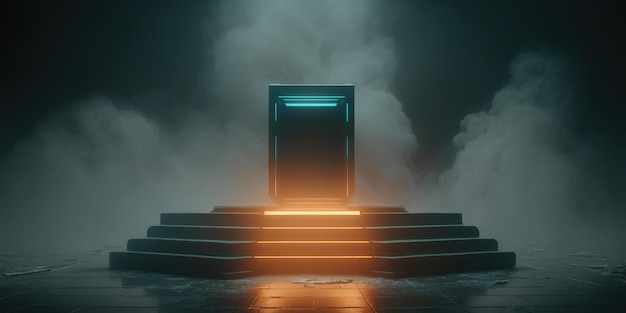The image depicts a surreal, movie-like set piece that appears futuristic and eerie. At the center of the scene is a set of four black-tiled stairs leading up to a small platform, on which stands a singular, closed door framed by a door frame. The door, although seemingly attached to nothing, suggests an entryway to another dimension or space. The background is engulfed in darkness and thick, smoky fog rising ominously behind the door and the stairs. There's a dramatic play of lights: a blue light emanates from behind the door, giving it an otherworldly glow, while a yellow LED strip illuminates the top stair, casting a pathway forward. The floor in front of the stairs shows faint reflections, possibly of water lapping at the base, adding to the surreal and foreboding atmosphere. The entire scene feels like a portal to an unknown, potentially ominous realm.